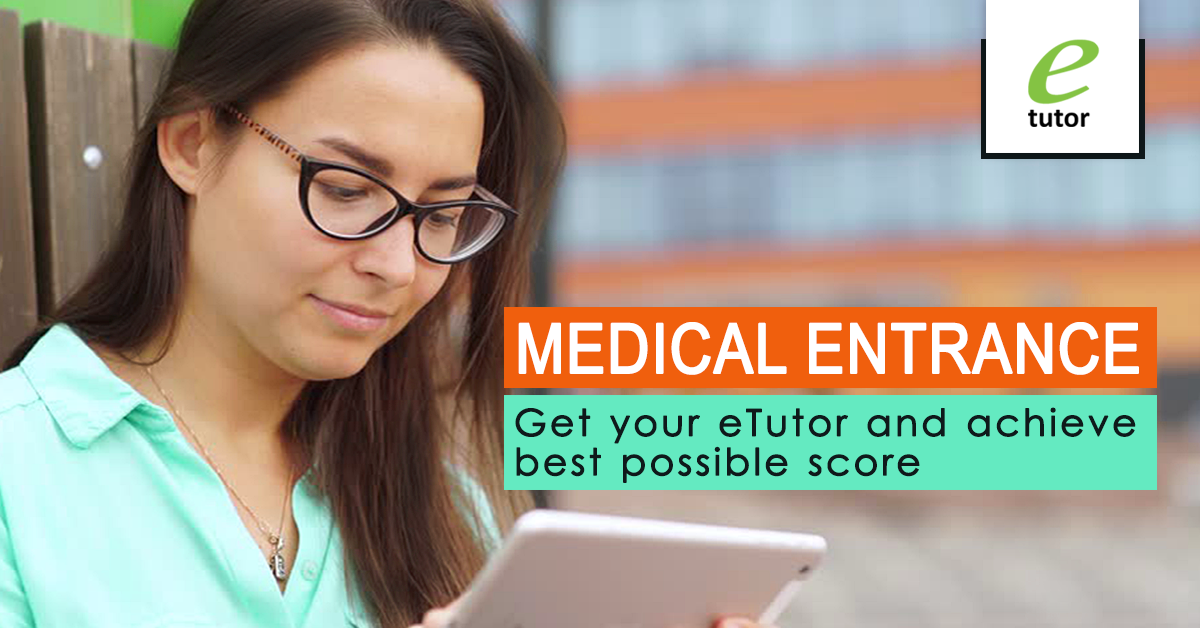This horizontal advertisement features a young woman occupying the left one-third of the image. She's depicted from the chest up, wearing dark-framed glasses, a light turquoise shirt, and a delicate necklace. Her long brown hair cascades down as she bends her head slightly, engrossed in reading something on her tablet or mobile device. She stands against a wooden fence, with green foliage or a green wall visible above the planks in the upper left corner.

The remaining two-thirds of the image on the right side are blurred, enhancing the focus on the woman. In the upper right corner, a small white square showcases a green letter 'E' followed by the word 'Tutor' in black. Centrally located on the right side, a rectangular block of text stands out with a segmented background of orange and turquoise. The text reads in light beige letters on an orange background: "Medical Entrance," followed by the message: "Get your e-Tutor and achieve best possible score," in black letters against a turquoise background.